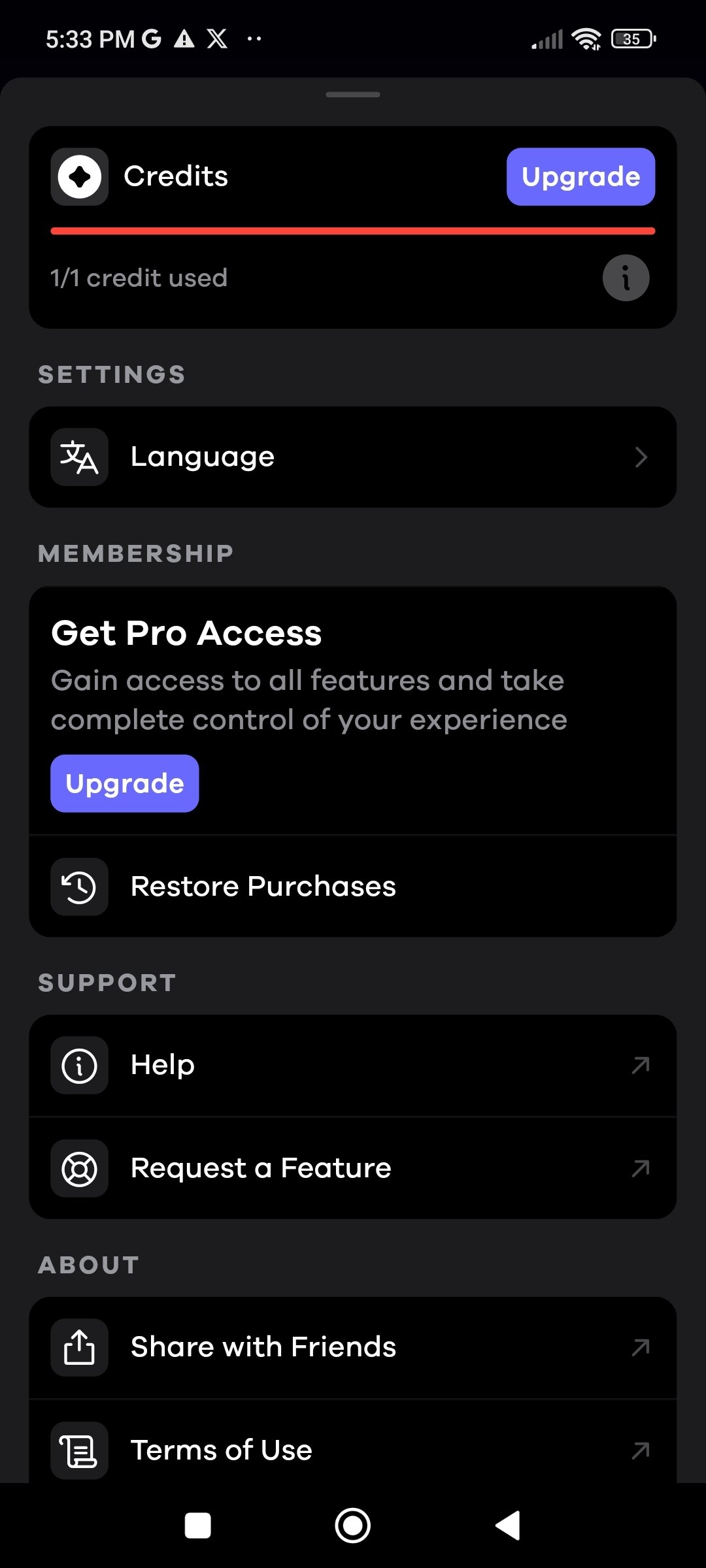The image is a screenshot of a smartphone in dark mode, featuring a predominantly black background. The top section of the screen displays the current time in white digits, reading 5:33 p.m. Adjacent to the time, icons indicate a "G," a triangle symbol, and an "X," suggesting the user is on Twitter. On the upper right corner, we can see icons for signal strength, Wi-Fi connectivity, and battery status, which shows 35% remaining.

Below this, there is a small rectangle banner. On the left in white text, it reads "Credits," and to its right, on a purple background with white letters, is the word "Upgrade." This banner is divided by a red line, and beneath it, it states "one-of-one credit used." What follows is a list of settings options:

- First, "Settings" is labeled, followed by a rectangle containing "Language."
- Next, "Membership" is indicated, underneath which another rectangle displays "Get Pro Access" in white letters.
- An explanatory text follows, "Gain access to all features and take complete control of your experience."
- Below this, another purple box with white letters reads "Upgrade."

Towards the bottom of the screen, an arrow forms a three-quarters circle pointing left, accompanied by the text "Restore Purchases." Finally, at the bottom, the word "Support" is seen inside another rectangle, containing the options "Help" and "Request a Feature."